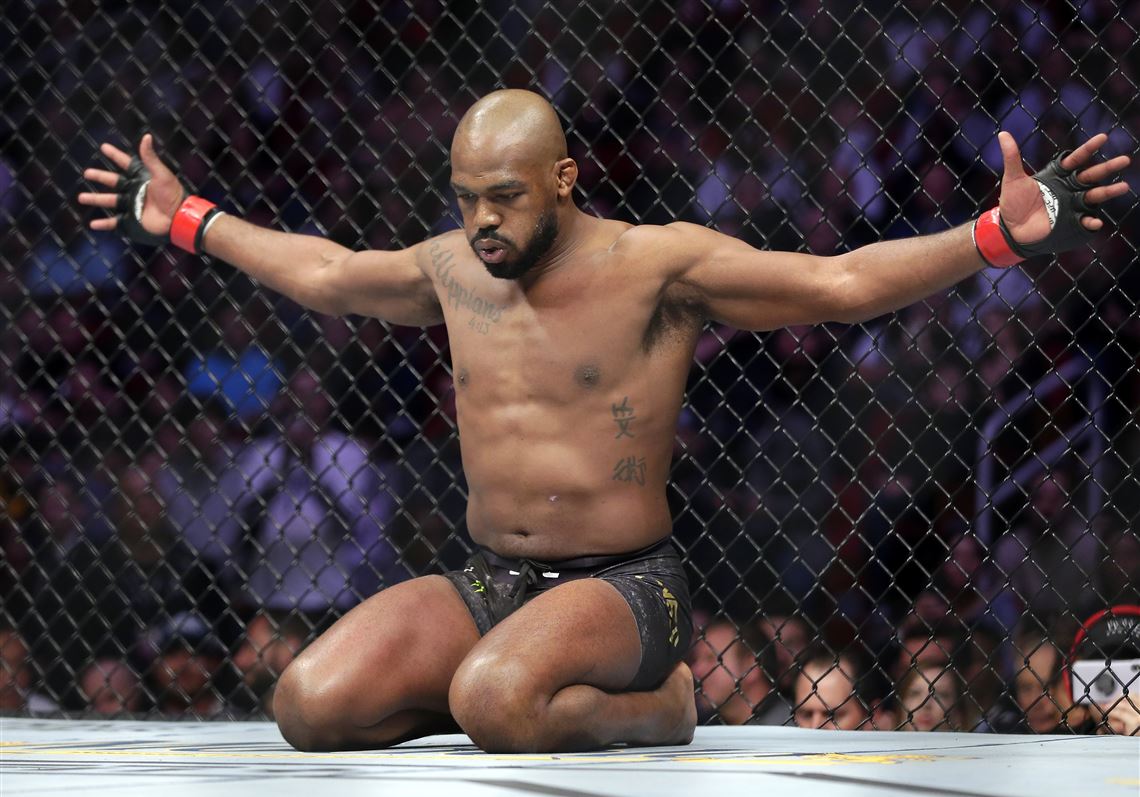A shirtless African American MMA fighter with a bald head and a beard is kneeling on a light-colored mat inside a fenced-in area of an athletic event, likely an MMA fight. He is wearing black shorts with yellow accents and black fingerless gloves with red wristbands. His body is adorned with tattoos in what seem to be Asian characters on his ribs, while additional text, including the numbers "413," can be seen on the upper right side of his chest. The fighter appears to be catching his breath, his arms outstretched and looking down with puffed lips as though in a moment of reflection or prayer. Behind the cage, spectators are packed into the stands, watching from both ground level and higher tiers. The scene is filled with an array of colors—blue, black, red, purple, gray, and brown—adding to the intense atmosphere of the event.